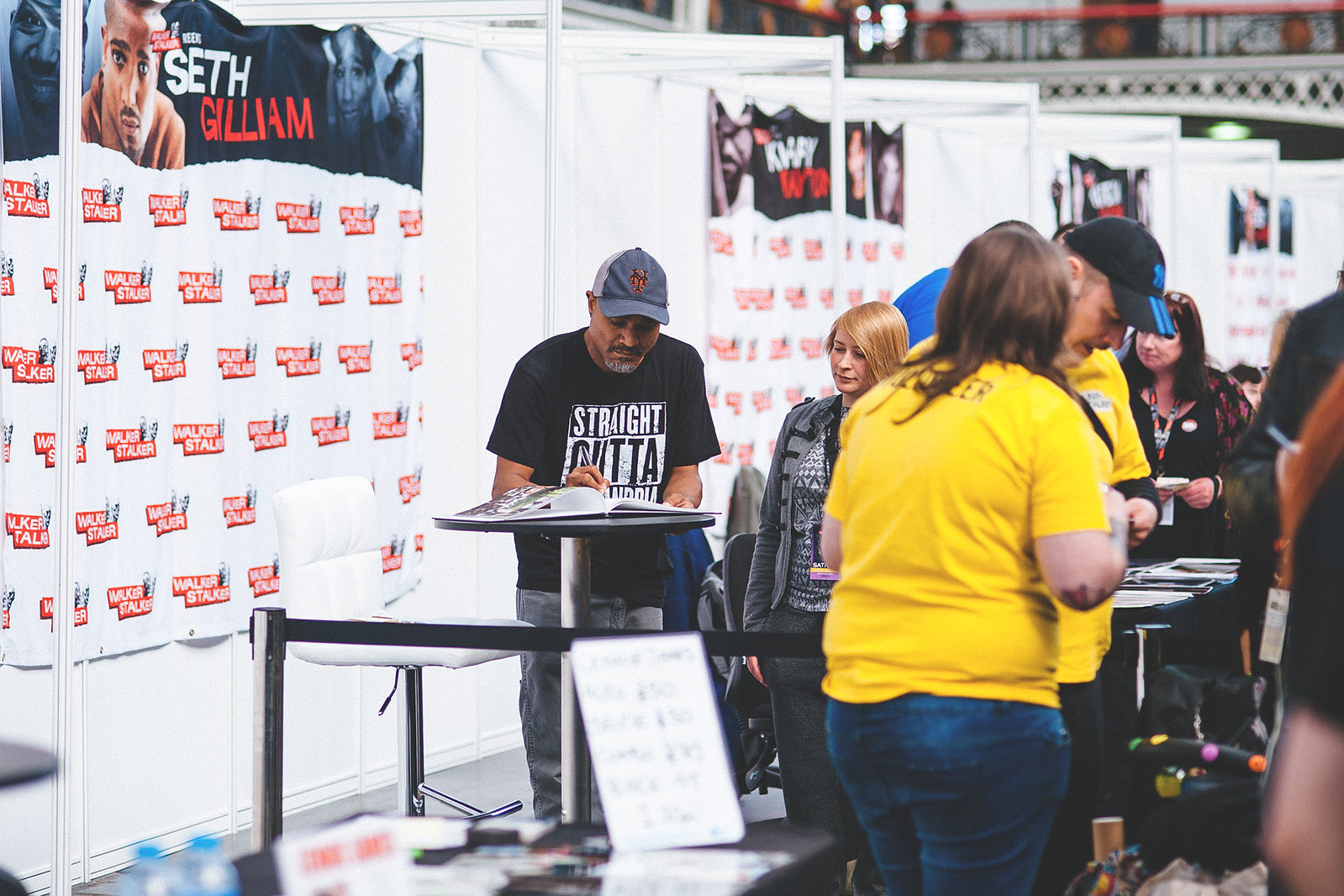At a vibrant convention, a central figure, Seth Gilliam, is positioned behind a sleek, silver podium with a round black top. Dressed in a black shirt emblazoned with "Straight Outta" and a light blue baseball cap, he leans over, signing an open book. Surrounding him is a lively scene; to his immediate right, a red-haired woman in a suit jacket with gray arms focuses intently on the book being signed. Further right, a woman in a yellow shirt and blue jeans, with dark brown hair reaching her shoulder blades, stands with her hands clasped. Nearby, a man's head, donning a dark black cap with blue lines, is bowed. The backdrop features a white wall adorned with banners, prominently displaying "Seth Gilliam" alongside his picture and the ubiquitous "Walker Stalker" convention logos, creating a bustling and energetic atmosphere indicative of a popular autograph session.